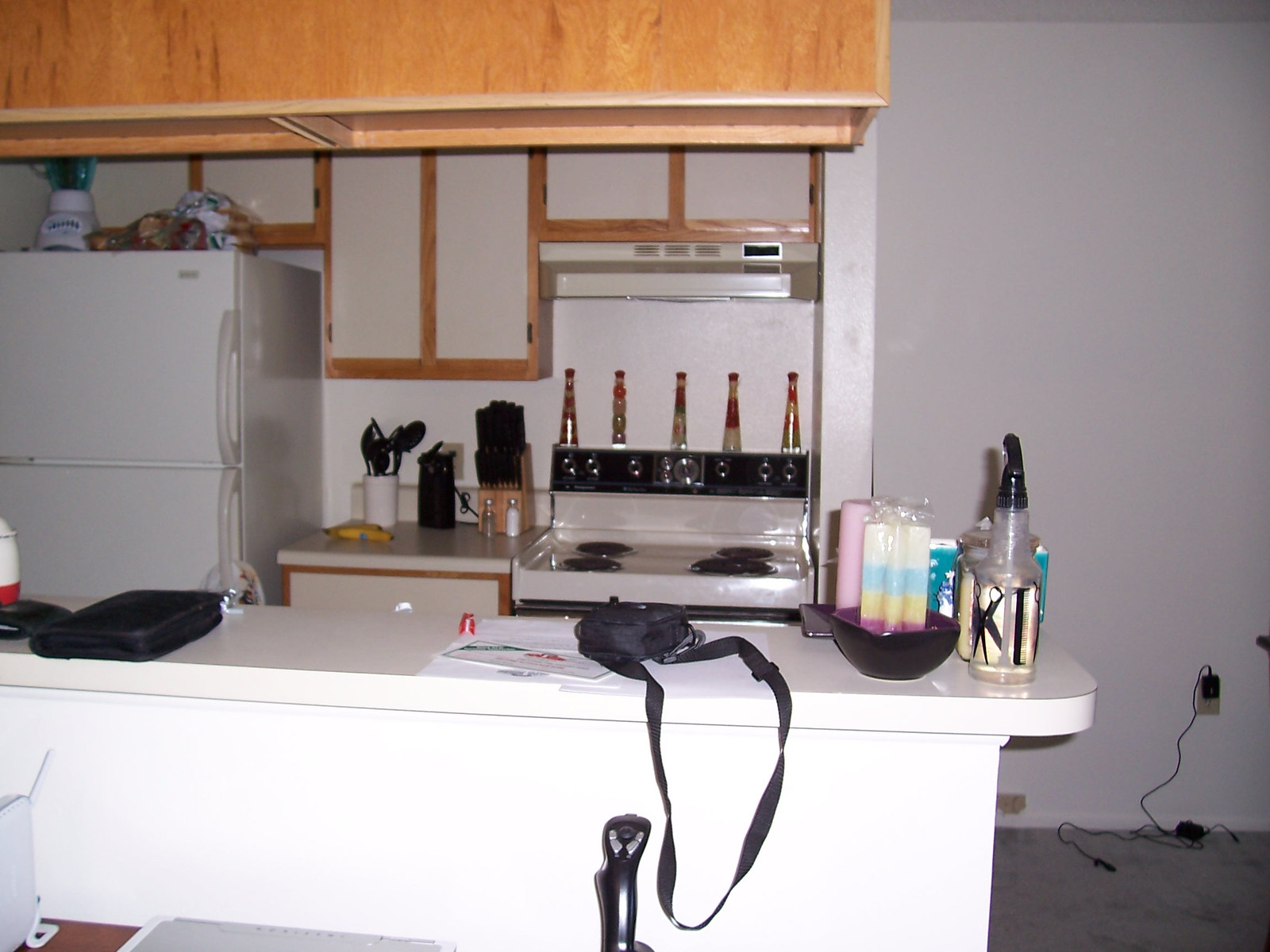This image captures a comprehensive view of a kitchen from the perspective of the adjacent room. Dominating the foreground is a white kitchen island, which serves as a boundary between the kitchen and the other room. The island features a pristine white countertop. On this countertop sits an array of items: a black bowl filled with various objects, a red and white water bottle or drinking container, a black zip-around case likely used for holding a book or CDs, and a spray bottle positioned to the right. Further down the island, a bag with a long black strap rests on a stack of papers with red and black lettering.

Behind the island, the left side of the kitchen reveals a white refrigerator, a freezer-over-fridge model with handles on the left for right-to-left opening. The top of the refrigerator is cluttered with bread and assorted food items. Adjacent to the fridge is a small section of tan countertop, which houses a white cylindrical vessel filled with black plastic kitchen tools including a spoon, slotted spoon, ladle, and whisk. Next to this vessel is a black electric can opener and a wooden knife block showcasing knives with black handles. In front of the knife block sits a clear glass salt and pepper shaker set.

To the far right is a black and white stove, identifiable by its array of knobs lined along its back. The stove is either adorned or accompanied by slender bottles, potentially containing vinegar or olive oil, further enhancing the functional and lived-in ambiance of the kitchen.